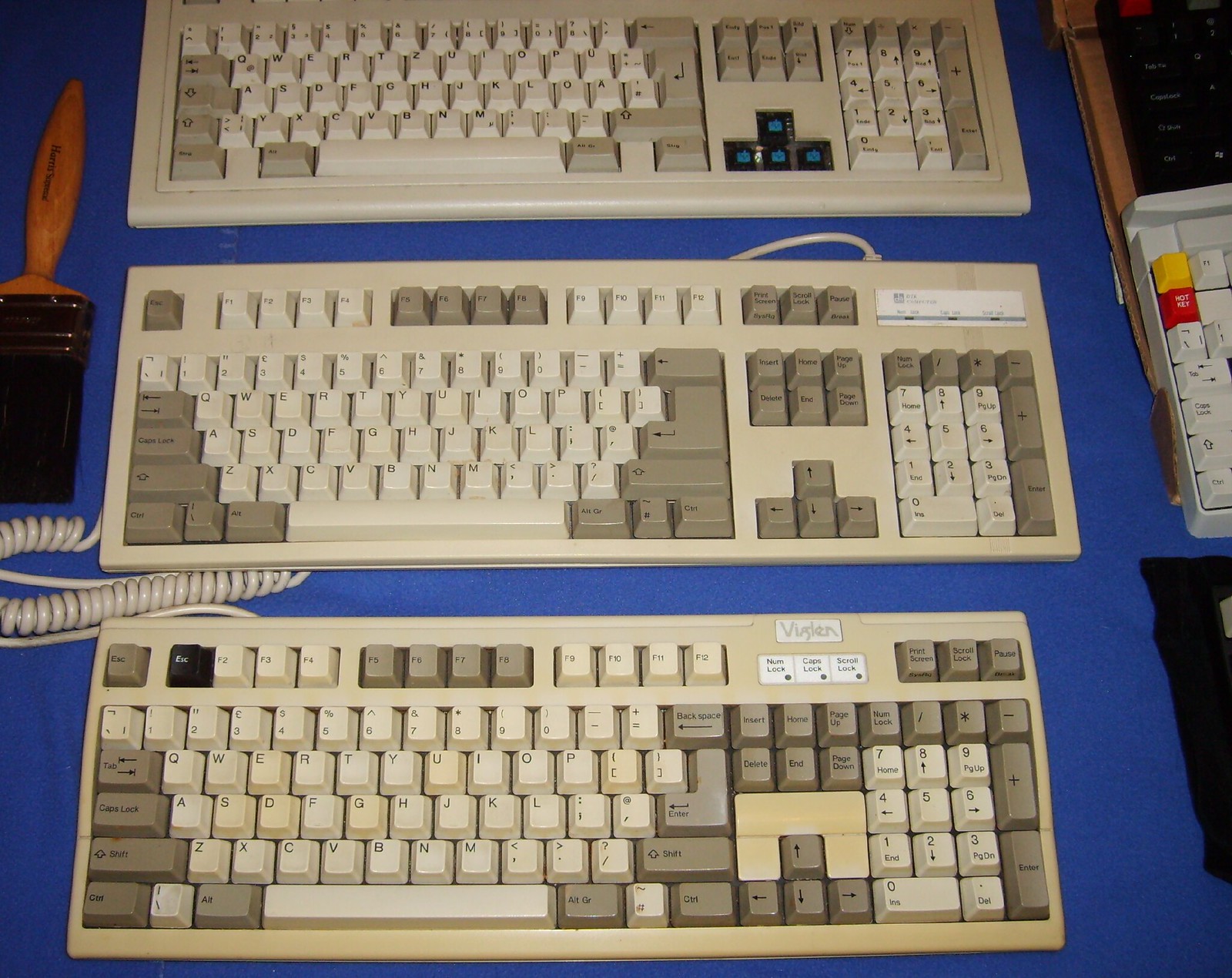The photograph features three vintage computer keyboards placed on a blue tablecloth. The keyboards, which are all cream or tan in color and show signs of aging with yellowed keys and components, vary slightly in their design and condition. 

The bottom keyboard, possibly branded as Vertin or Vision, is the oldest. It has noticeably yellowed keys which appear worn and hard to press, and features a cord attachment. The middle keyboard is slightly newer, still has a cord, and exhibits less yellowing on the keys but has a yellowed baseboard with something taped in the upper right-hand corner. A paintbrush with its bristles down is positioned to the left of this keyboard.

The top keyboard is the newest among the three. It is the cleanest with lighter, less yellowed colors and features black arrow keys with blue markings. Notably, it does not have an attached cord. Additionally, to the right side of the photograph, the edges of other keyboards or possibly a nine-key adding machine can be seen. Overall, the image captures the gradual evolution of keyboard designs and their deterioration over time.